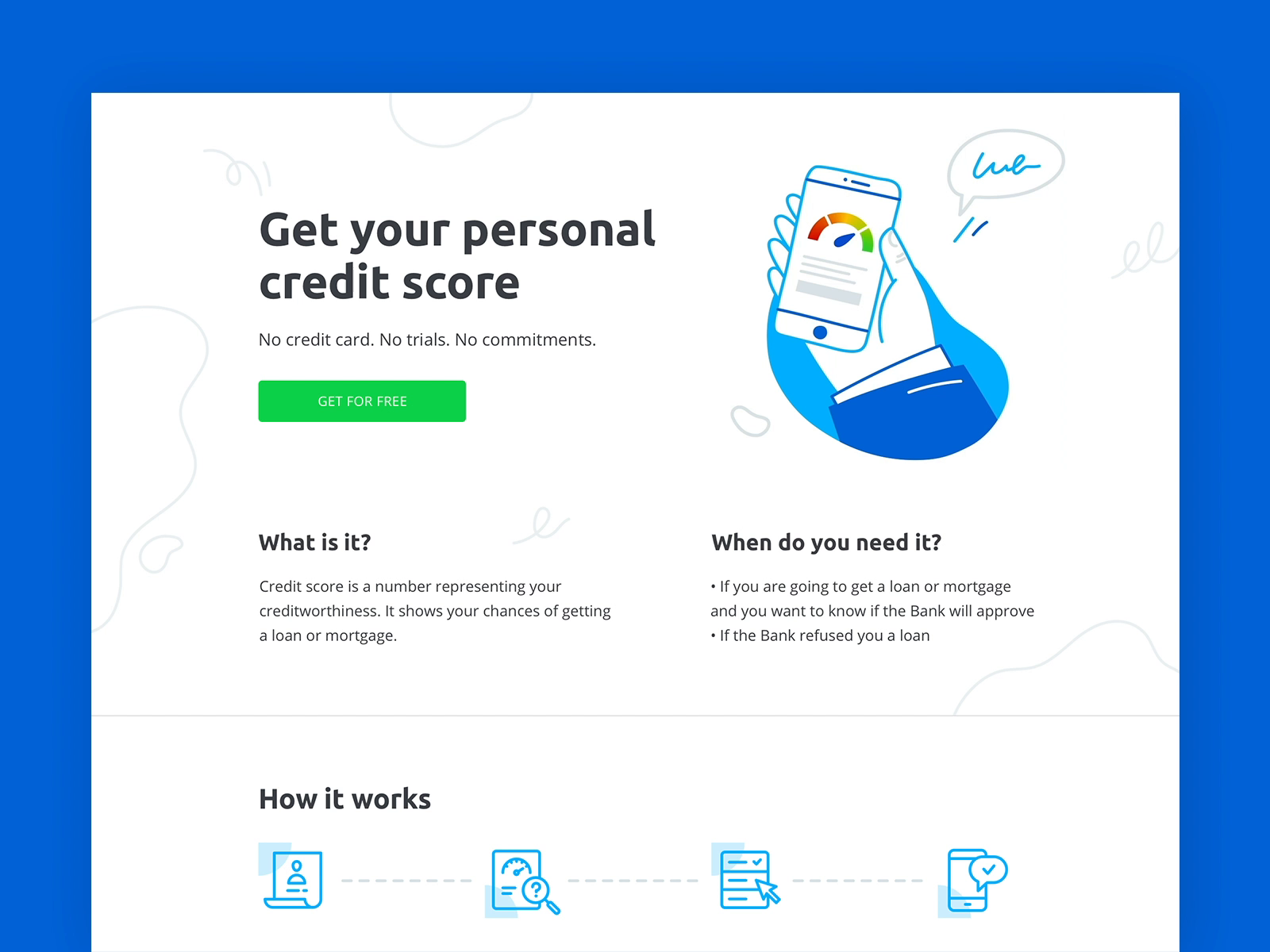The image displays a splash screen of a website designed for obtaining personal credit scores. On the right side of the screen, there's an illustrated hand holding a smartphone, which features a barometer-like gauge depicting the user's credit score. To the left, bold black text on a white background reads "Get Your Personal Credit Score." Below this, supportive text states, "No credit card, no trials, no commitments, get for free." This message is accompanied by a prominent green button with white text that says "Get for Free."

Beneath this call-to-action, there's an explanatory section addressing two key questions: "What is this?" and "When do you need it?" This text explains that a credit score is a numerical representation of one's creditworthiness and details its importance in scenarios such as obtaining loans or mortgages. It's clearly stated that understanding one's credit score can influence the approval of financial applications.

A fine gray line separates this upper section from a series of four blue and white icons at the bottom. These icons visually illustrate the process of how the credit score is generated.